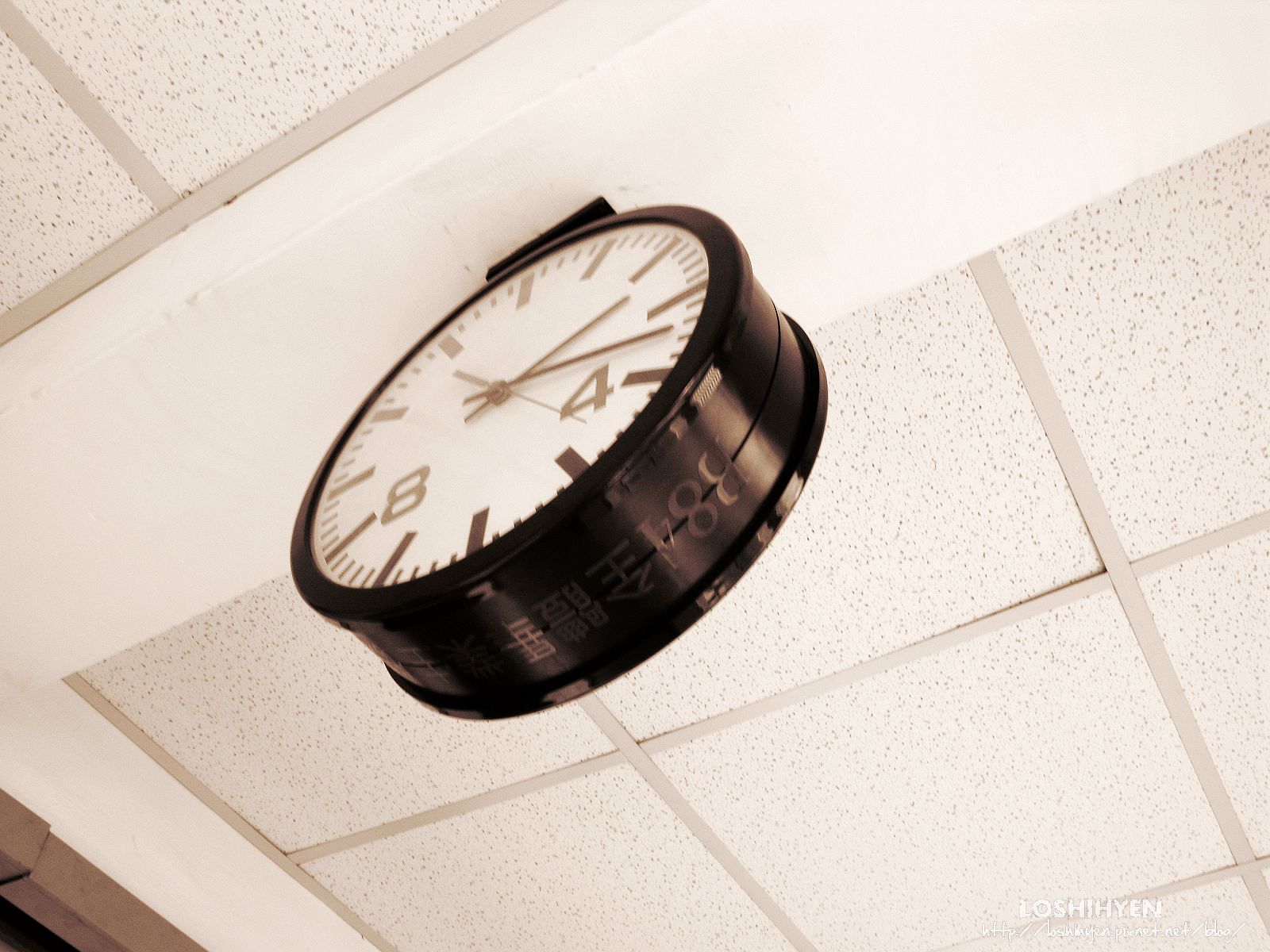The photograph is an indoor shot taken at a steep upward angle, focusing on a suspended clock near the ceiling. The ceiling is covered with light, airy, white soundproofing tiles featuring small holes. A prominent white beam extends diagonally from the mid-left to the upper right of the frame, supporting the metallic-looking clock. The clock itself has a shiny, possibly bronze or black circumference, its color dependent on the lighting. Its face is white with two prominent numbers, 4 and 8, while the other positions are indicated by solid black lines. The clock shows the time as 2:17, with the hour hand just past the 2 and the minute hand at 2 minutes past the 3. The clock, an old-style analog, also features a second hand. On the bottom, subtle silver reflective script includes the text "B8-4" along with some Japanese or Chinese characters. A piece of wood is descending diagonally from the bottom left, providing a sense of the commercial environment in which this clock is situated.